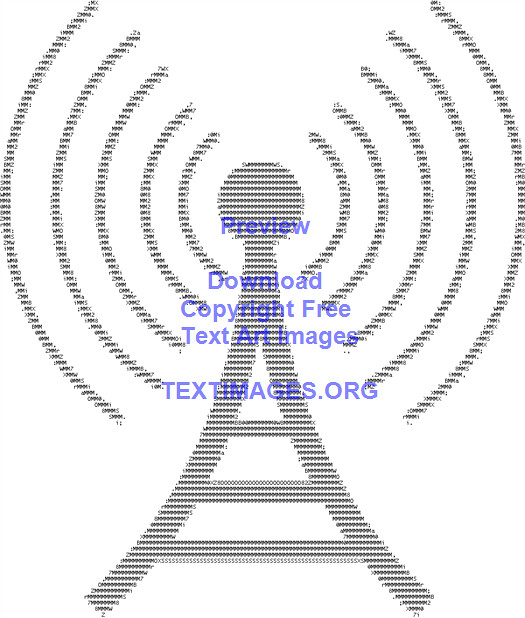The image showcases a detailed piece of ASCII art, an old form of digital art dating back to the 1980s and early 90s, meticulously crafted from various alphanumeric characters and punctuation marks. It depicts a radio tower, with a distinct circle in the middle and five rounded signals radiating from each side, simulating wireless signals. The entire image is composed of dense arrays of characters like S’s, M’s, numbers, and other symbols, showcasing the clever utilization of text to form a coherent and recognizable image. The background is stark white, making the intricate character work stand out. Overlaid on the image in bold purple text are phrases such as "Preview," "Download copyright free," "Text art images," and the website "textimages.org" in capital letters, urging viewers to download similar content from the specified site.